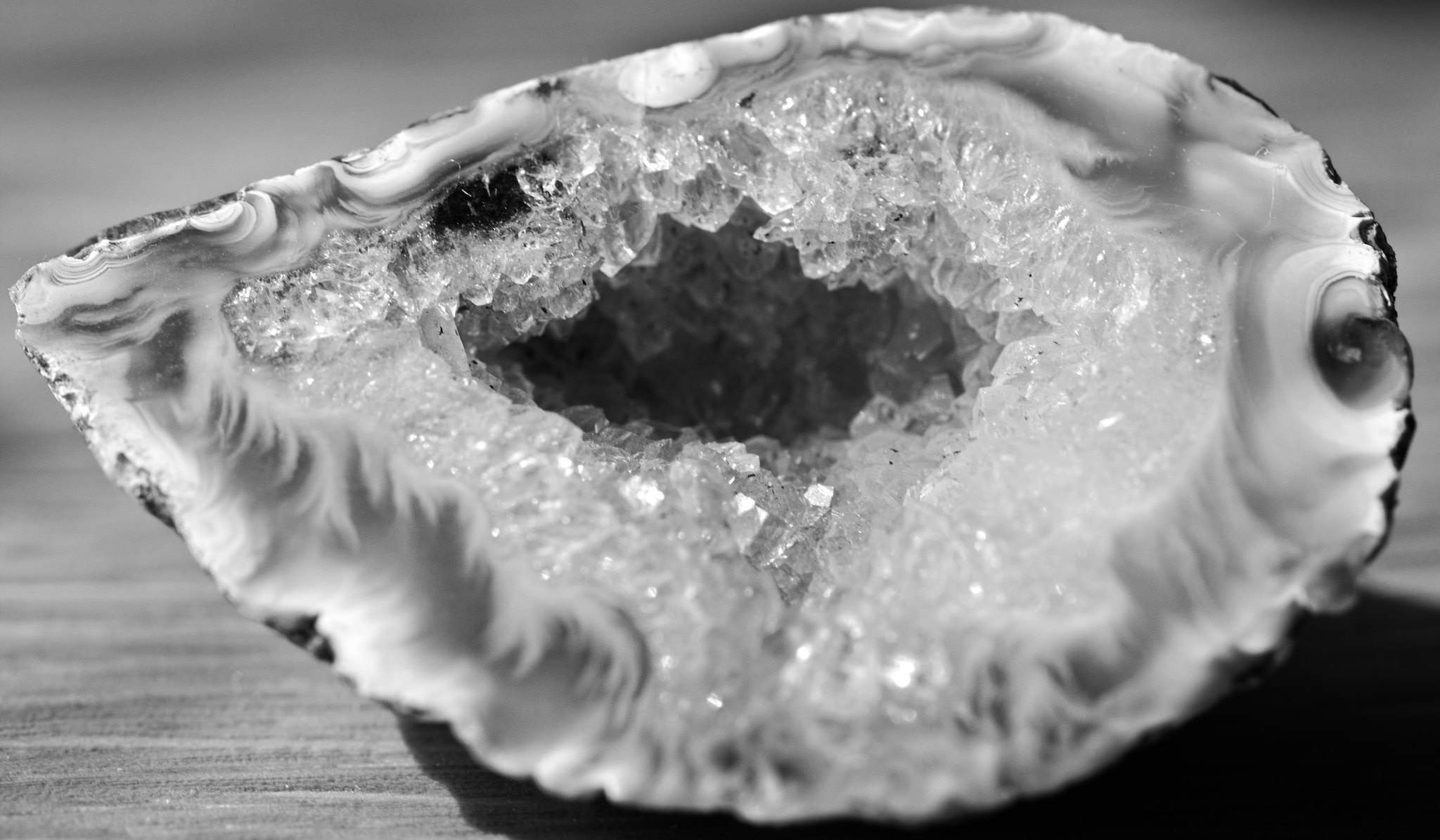This black-and-white photograph captures a detailed image of a teardrop-shaped geode, which has been cut in half, revealing its intricate interior. The geode, resembling an oyster shell, features a rough, dark exterior juxtaposed against a smooth, white perimeter that appears almost like a delicate paste. The focal point of the image is the central cavity filled with clear, transparent crystals, akin to a pile of caviar nestled within the geode's confines. The stark contrast between the outer and inner surfaces highlights the geode's natural beauty. Positioned on a wooden table with visible wood grain, the geode casts a shadow in the bottom right corner of the image, adding depth to the composition. Blurring in the top half of the photograph emphasizes the geode itself, providing a clear, textured view of its crystalline center. Notably, squirrels are positioned around the perimeter of the photo, adding an unexpected element to the scene.